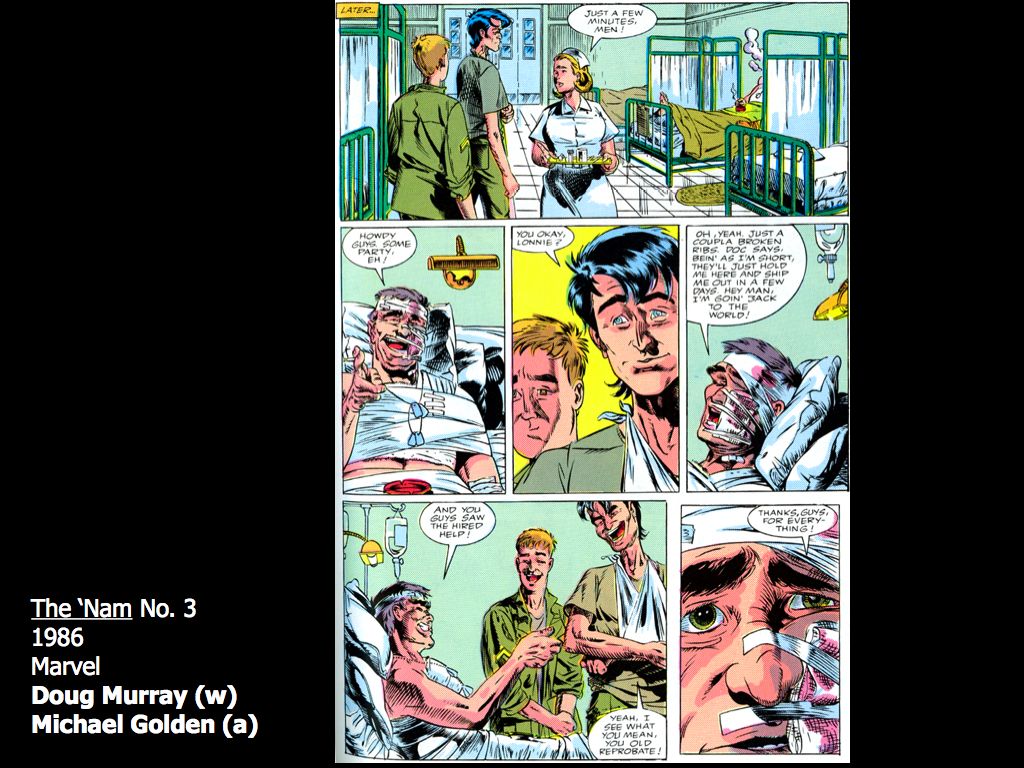This image is a detailed photo of a page from a comic book, set against a solid black background. In the bottom left corner of the image, the text reads: "The Nam, No. 3, 1986, Marvel, Doug Murray (W), Michael Golden (A)." The comic strip is arranged in three rows, each depicting scenes from a hospital setting in full color. The characters featured are two men, a woman nurse, and a patient. The top row shows two men and a nurse standing near hospital beds. In the second row, there is a close-up of a man lying in a hospital bed with his head bandaged, followed by a close-up of the faces of the two men standing. The bottom row includes a wider shot of the patient conversing with the two men, and a close-up of the patient's heavily bandaged face. The color palette of the comic page includes black, white, pink, tan, gray, red, green, yellow, and blue. Text bubbles indicate dialogue, but the small size makes them difficult to read. The comic page itself is centered within the image, resembling a page extracted from a comic book.